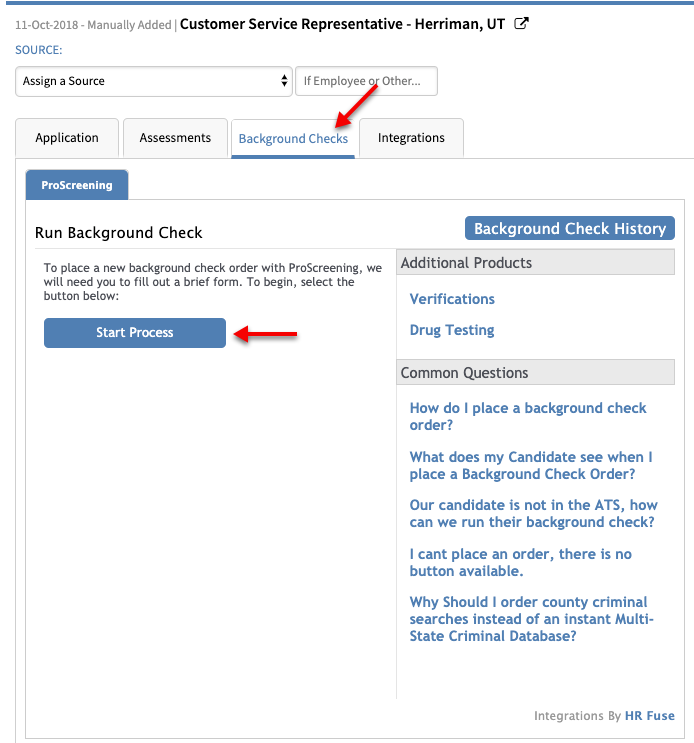The website's employee screening page presents a comprehensive interface for managing background checks. At the top, a thin blue line underscores the header, which includes the text "11-OCT-2018 - manually added" in gray, followed by "Customer Service Representative - Herriman, Utah" in bold black letters. Beneath this, the word "Source:" is presented in blue, accompanied by a box labeled "Assign Source" and another box that reads "If Employee or Other..."

The top section features four primary navigation tabs: "Application," "Assessments," "Background Checks" (highlighted in blue with a red arrow pointing to it), and "Integrations." Below these tabs is a prominent blue box titled "Pro Screening" in white text. Adjacent to this is a command box in black stating "Run Background Checks," with another blue box on the right labeled "Background Check History."

Further details on the page explain the process for placing new background check orders with Pro Screening. The instructions, in black text, state: "To place a new Background Check order with Pro Screening, we will need you to fill out a brief form. To begin, select the button below." Following this explanation is a blue button that says "Start Process" accompanied by a red arrow.

On the right-hand side of the page, there is a vertical column of headers and questions. Starting with "Additional Products," the section includes options like "Verification and Drug Testing" in blue. Below this header, the "Common Questions" section provides answers to frequently asked questions such as "How do I place a Background Check order?", "What does my candidate see when I place a Background Check order?", "Our candidate is not in the ATS, how can we run their Background Check?", "I can't place an order, there is no button available," and "Why should I order County Criminal Searches instead of an Instant Multi-State Criminal Database?" The bottom of the column features the integration tool "H.R. Fuse."